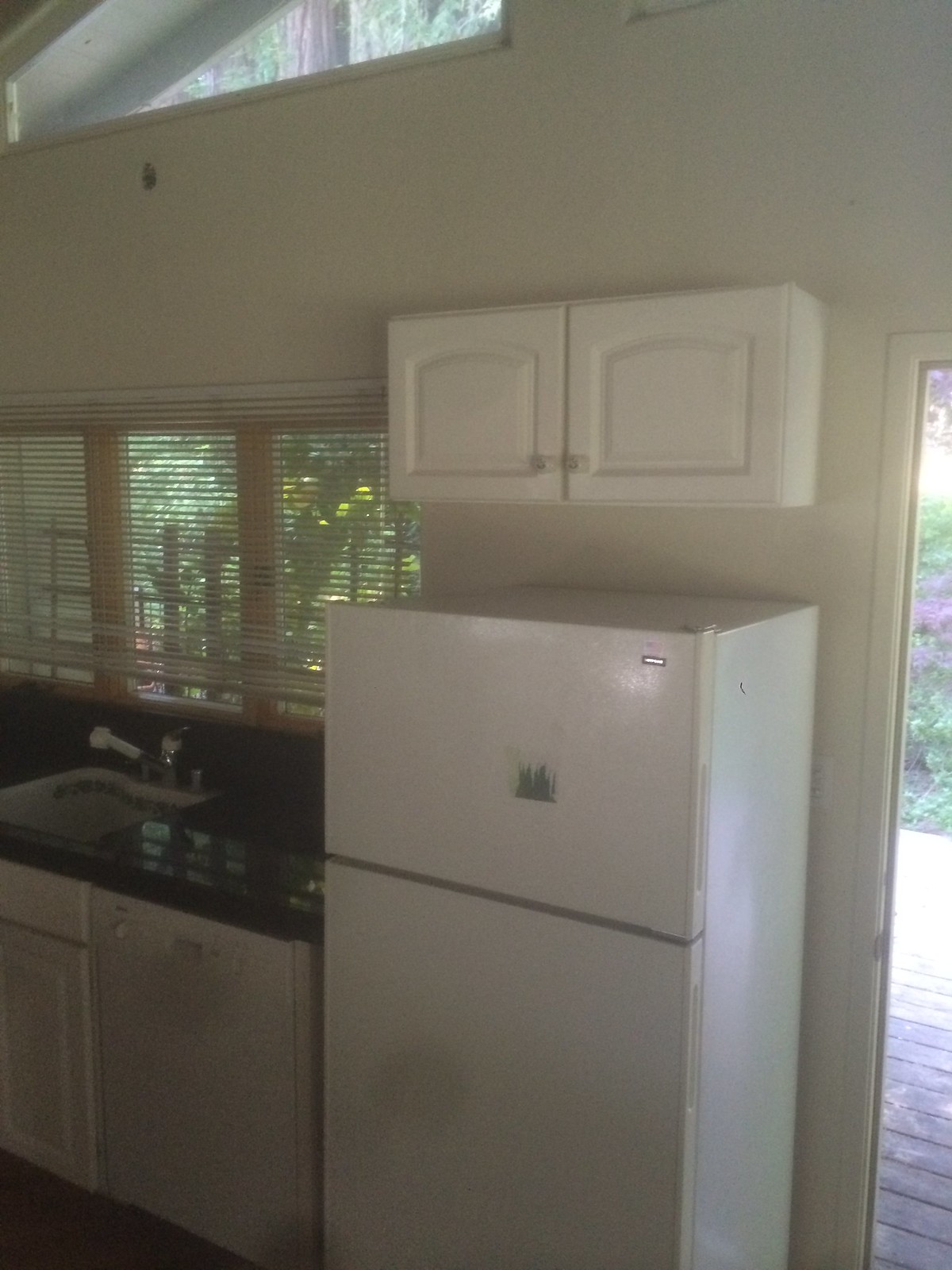This color photograph, taken in a low light setting, captures the interior of a home kitchen, highlighting a white refrigerator with a top freezer positioned front and center. Above the fridge, there's a white cabinet with two doors. To the left of the fridge, under a window covered by vertical blinds, stands a white dishwasher integrated into the black countertop. The sink is situated next to the dishwasher, with more windows above it. High ceilings accentuate the space, featuring a triangular window on the top left side. Adjacent to the kitchen is a glass door that leads to the backyard, revealing wooden decking, greenery, and purple flowers. The kitchen's black countertops contrast with the white cabinetry, creating a sleek and functional environment. The slightly grainy quality and portrait orientation of the photograph further add to its residential charm.